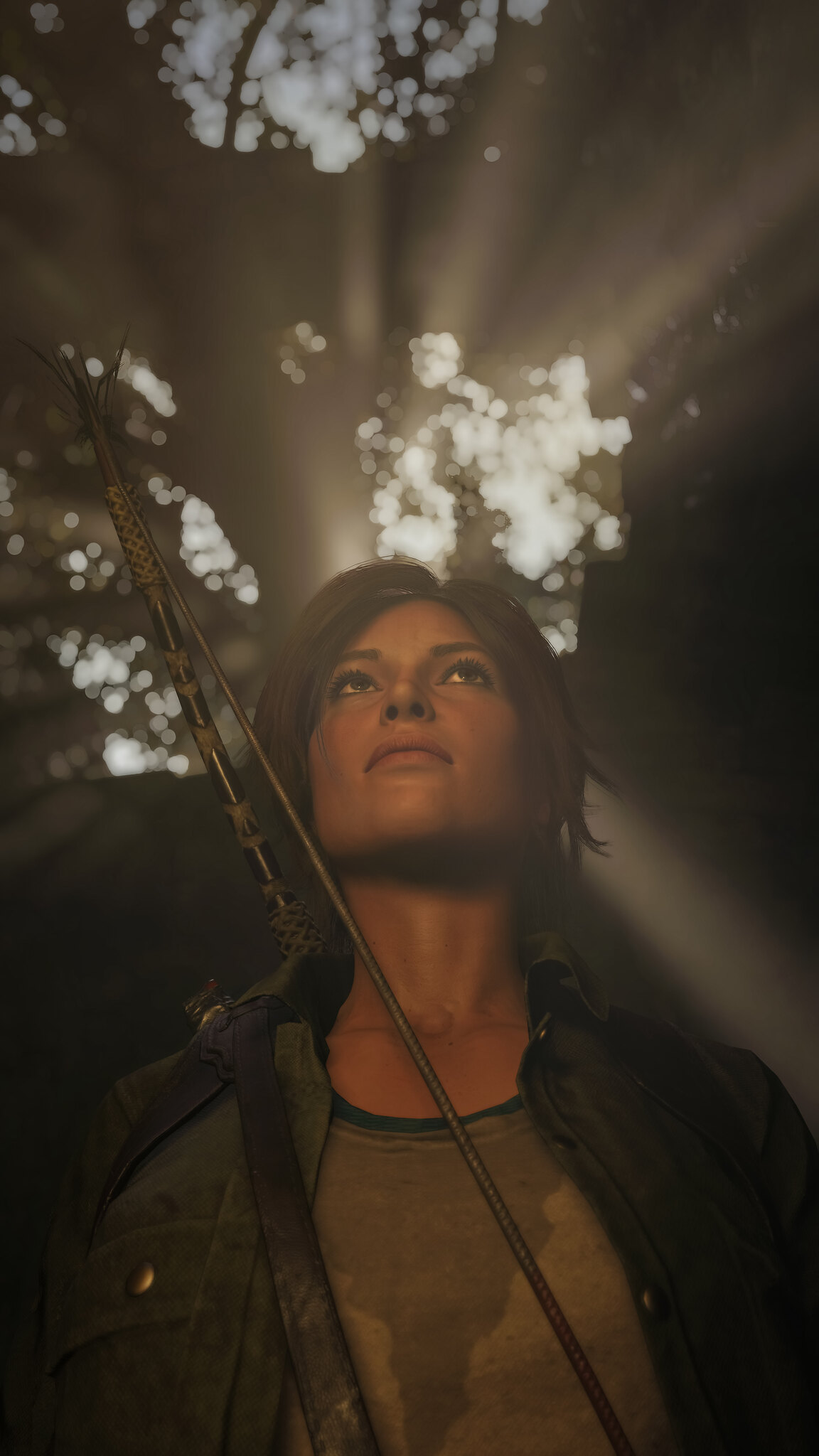In this realistic photograph, reminiscent of a cinematic screenshot or a video game still, we see a woman standing in the foreground beneath a canopy of trees that form a circular opening to the sky. Rays of sunlight filter through the trees, casting visible light beams behind her. The woman has chin-length brown hair and a fair complexion. She is gazing upwards, looking straight ahead with a calm expression. She wears a long-sleeved denim jacket over a gray shirt that is visibly sweat-stained. A dark-colored bow, possibly black or dark brown, is wrapped around her, with the strap encircling her shoulder and the bow's limbs visible across her head and back. The intricate background of blurred leaves and trees enhances the image's serene and reflective mood, accentuated by the striking sunlight filtering through.